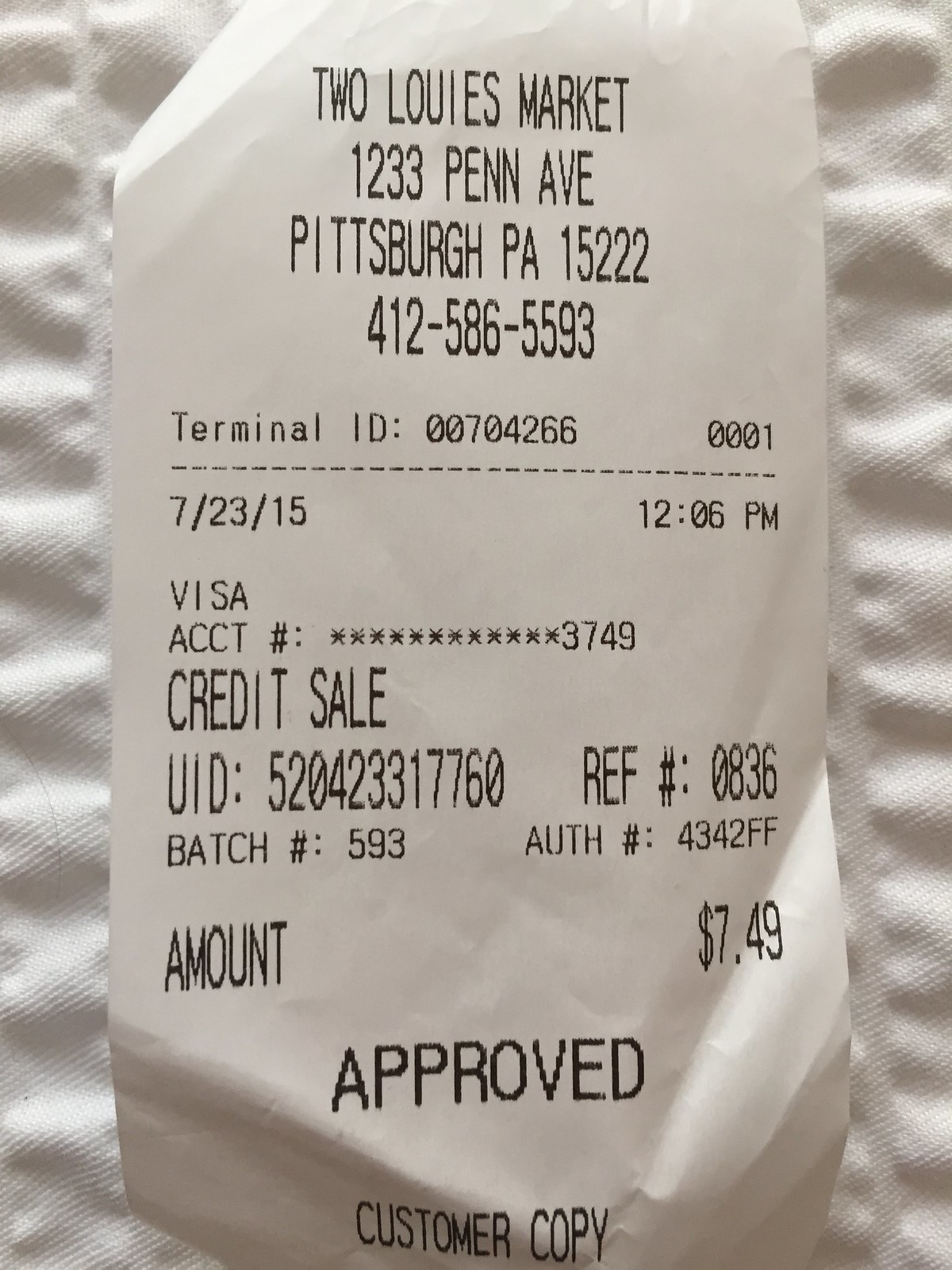The image captures a detailed close-up of a customer receipt from Louie's Market, located at 1233 Penn Avenue, Pittsburgh, PA 15222. The receipt, printed in black lettering on thin white paper, is displayed against a white textured background that resembles an enlarged paper towel. Key details shown include the store's phone number, 412-586-5593, and terminal ID, 00704266. The transaction took place on July 23rd, 2015 at 12:06 PM, using a Visa card ending in 3749 for a credit sale totaling $7.49, which was approved. Additional identifiers include the batch number 593, authorization number 4342FF, UID 520423317760, and reference number 0836. Notably, the receipt is marked as the customer copy.